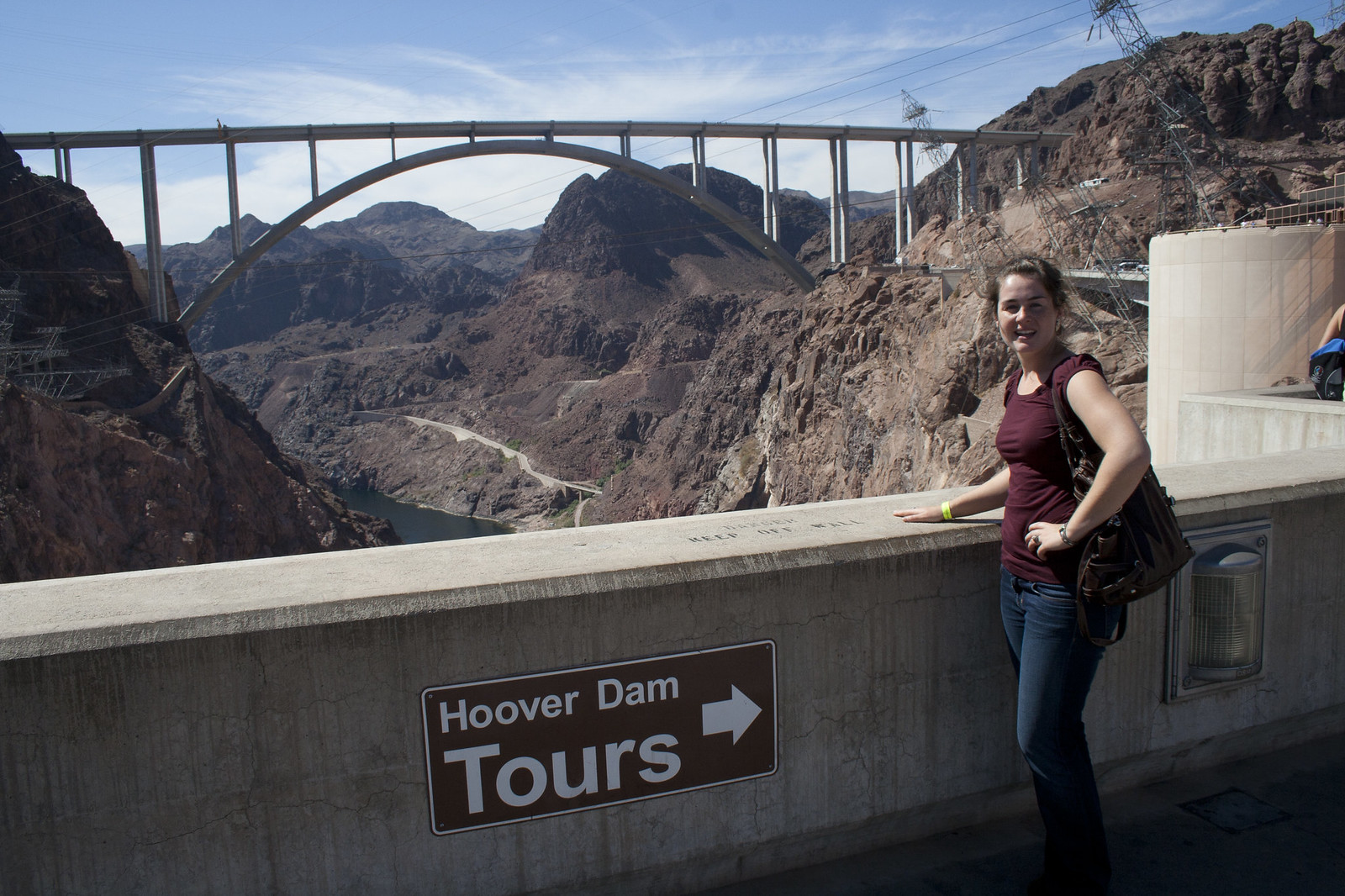In this image, a young woman with brunette hair stands beside a concrete wall adorned with a brown sign, bordered in white, that reads "Hoover Dam Tours" with an arrow pointing to the right. She is wearing a short-sleeved maroon top, blue jeans, and a lime green bracelet, with a leather brown bag slung over her shoulder. Her right hand is gently resting on the wall as she faces the left, turning her head towards the camera with a bright smile. Behind her stretches the vast expanse of the Hoover Dam area. The scene includes a glimpse of the river far below, partially obstructed by the massive structure of the dam. The Pat Tillman Memorial Bridge can be seen spanning rocky cliffs in the background, with power lines and angled electrical towers on the hillside. Additionally, cranes, a white tower, and other visitors populate the background under a clear sky.